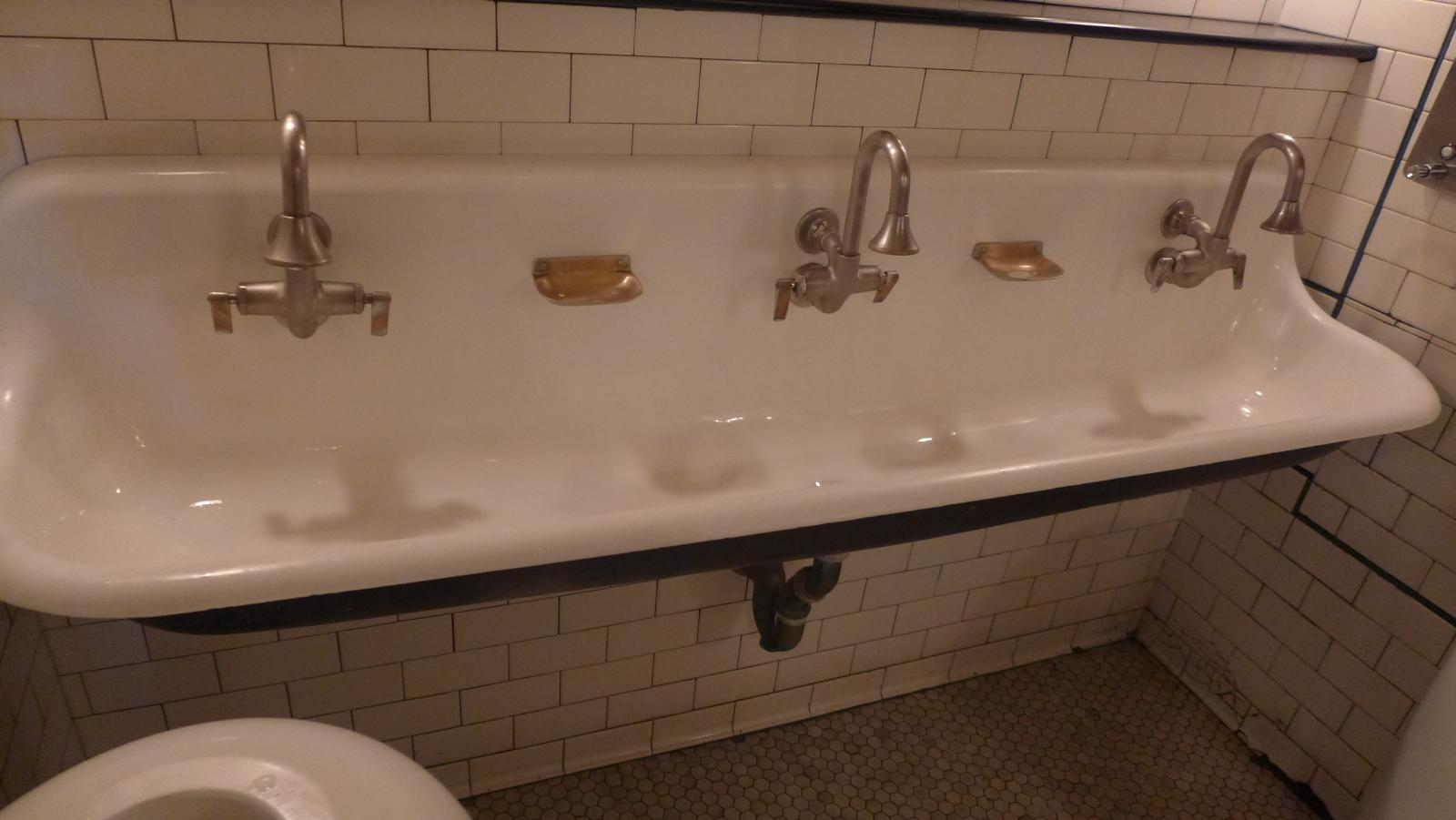The photograph depicts a slightly grimy public school bathroom with a distinct vintage vibe. It features a horizontally cropped image with a visible white porcelain sink that stretches remarkably long, bordered by a white tile wall with aged cream-colored grouting. Three industrial-looking silver faucets, each equipped with flip levers, are evenly spaced across the sink. Between each faucet, there's a copper-colored soap holder, maintaining a sequence of faucet-soap holder-faucet-soap holder-faucet. The sink's underside reveals a hefty steel drain pipe coursing centrally, contrasted by a backdrop of subway tiles that extend around and to the right of the sink. In the bathroom’s lower left-hand corner, a white barrel-shaped plastic trash bin with a hole at the top peeks into view. The floor consists of worn tiles patterned in gray and brown circles, appearing especially filthy in the corners, further accentuated by the pinkish-red lighting cast over the scene.